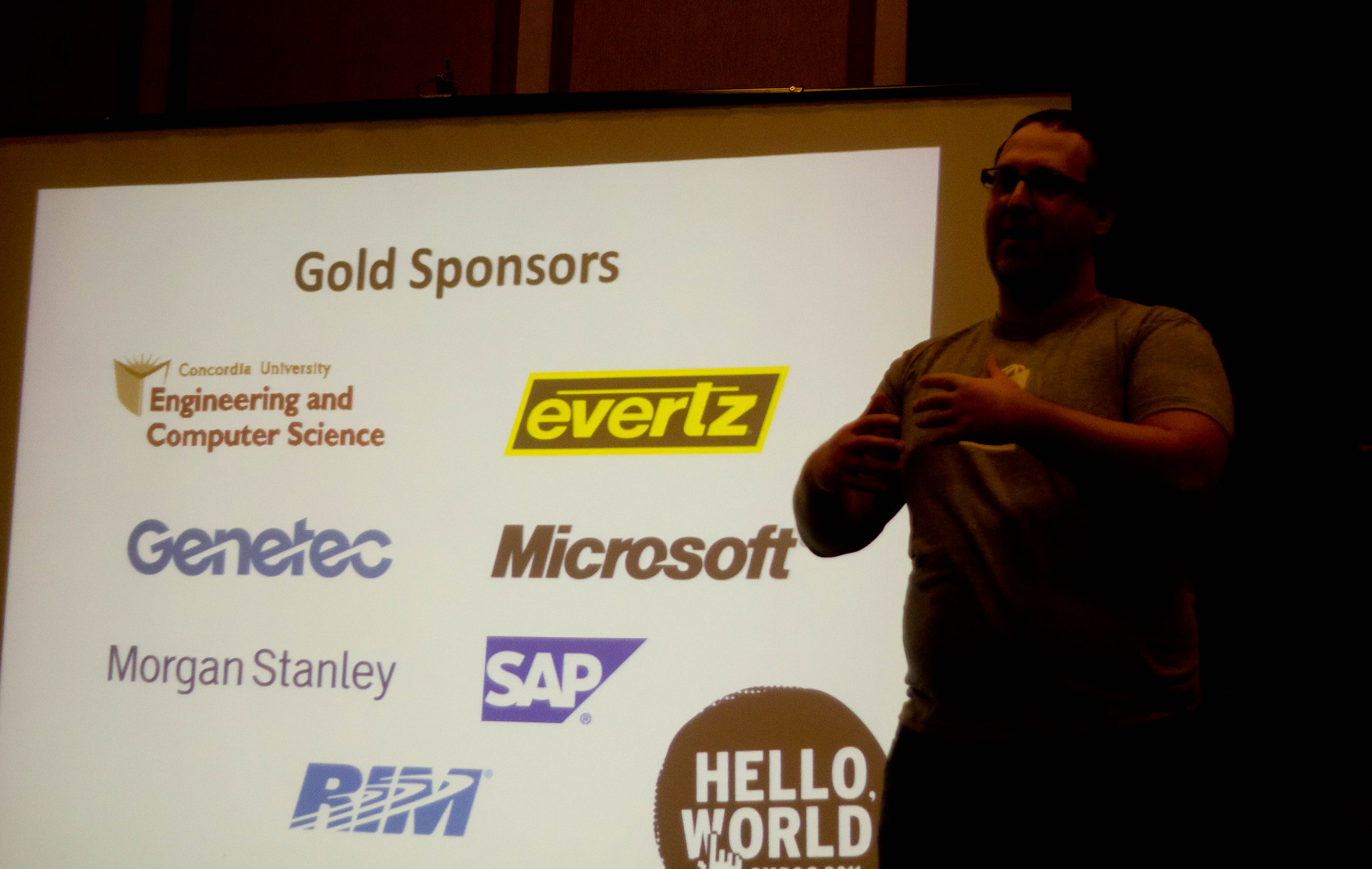A man with short dark hair and glasses is standing on the right side of the image, partially illuminated by the light from a projection screen next to him. He has a muscular build and is wearing a dark t-shirt with a symbol on the chest, which appears to be obstructed by his hands as he makes a gesture in front of his chest, likely while explaining something. The background behind him is dimly lit, casting him in shadow. The projection screen has a white background displaying several logos and text. At the top of the screen, center-justified black text reads "Gold Sponsors." Below that, the listed sponsors include Concordia University, Engineering Computer Science, Genetech, Morgan Stanley, Ivetz, Microsoft, SAP, RIM, and Hello World.